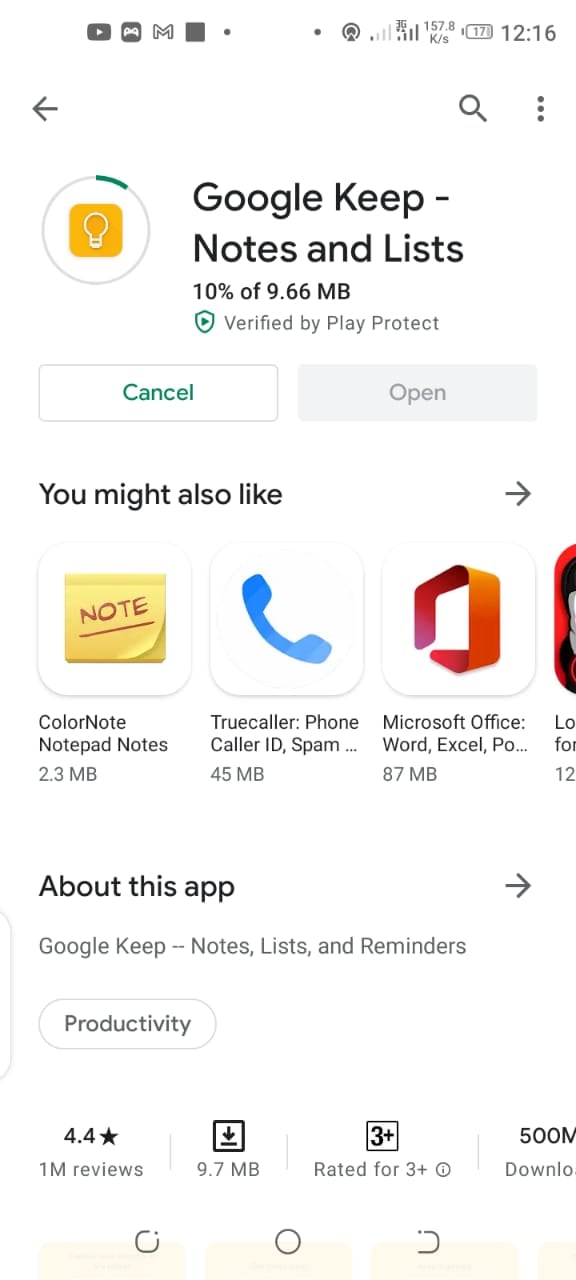**Description:**

A screenshot of the Google Play Store on a mobile device.

**Details:**

- **Top Bar (Left to Right):**
  - Gray YouTube icon.
  - Controller icon with a white controller on a gray square background.
  - Gmail logo.
  - Gray square icon.
  - Gray bullet point.
  
- **Upper Section:**
  - Top left corner has a gray left-pointing arrow.
  
- **Main Content:**
  - An app in the process of downloading:
    - **Icon:** Yellow with rounded corners featuring a white outlined light bulb.
    - **Progress Indicator:** Light gray border with a green area at the top showing download progress.
    - **App Name & Description:** "Google Keep - Notes and Lists" in black text.
    - **Download Progress:** "10% of 9.66 MB" downloaded.
    - **Security Verification:** Green shield with "Verified by Play Protect" in gray text.
  
- **Buttons:**
  - **Cancel Button:** Light gray border, white background, "Cancel" in green text (enabled).
  - **Open Button:** Light gray background, "Open" in gray text (disabled).

- **Suggestions Section:**
  - Header: "You might also like" in black text.
  - Listed App Icons:
    - "ColorNote Notepad Notes"
    - "Truecaller: Phone Caller ID, Spam"
    - "Microsoft Office: Word, Excel, Po…"